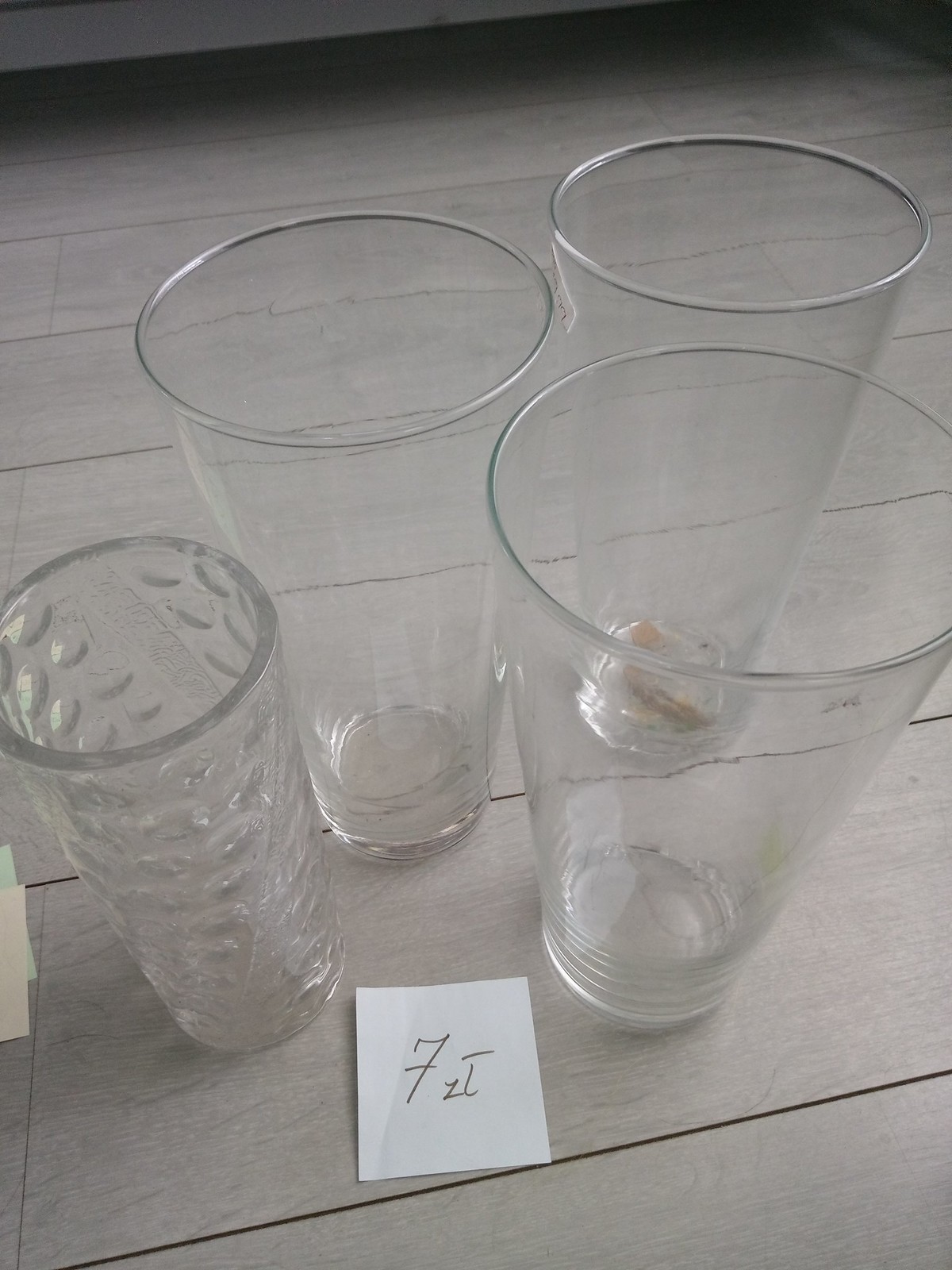This image captures a light grayish wood table, possibly artificial wood, with four empty drinking glasses positioned centrally in a slightly overhead view. Three of the glasses are of the same type, each wider at the top and tapering towards the base. The glass on the left is distinct from the others, featuring a textured, thicker design and tapering shape. It resembles a mojito glass and is wider at the top, tapering downward. Next to it, the two matching glasses are lined up side by side. On the right, another glass, also transparent and of the same height as the first pair, contains a remnant of a brown drink. Beneath one of the glasses is a small white piece of paper with the text "FZT," although part of the note is obscured, making it difficult to fully discern the additional markings.